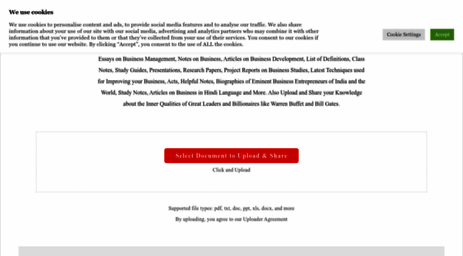The image features a visual layout commonly seen in website cookie consent banners. At the very top, bold black letters declare, "We Use Cookies." Directly below this, a paragraph in standard black print begins with, "We Use Cookies," but the font size is so small that the rest of the text is illegible. Further down, there is another paragraph in black print, characterized by slightly more spaced-out lines, though the text remains too small to decipher. Beneath this text block, a red rectangular button contains white text, typically indicative of an action prompt like "Accept" or "Learn More." Finally, at the bottom of the image, additional black text is placed above a gray rectangle that spans the width of the image, likely serving as a footer or an additional call to action.